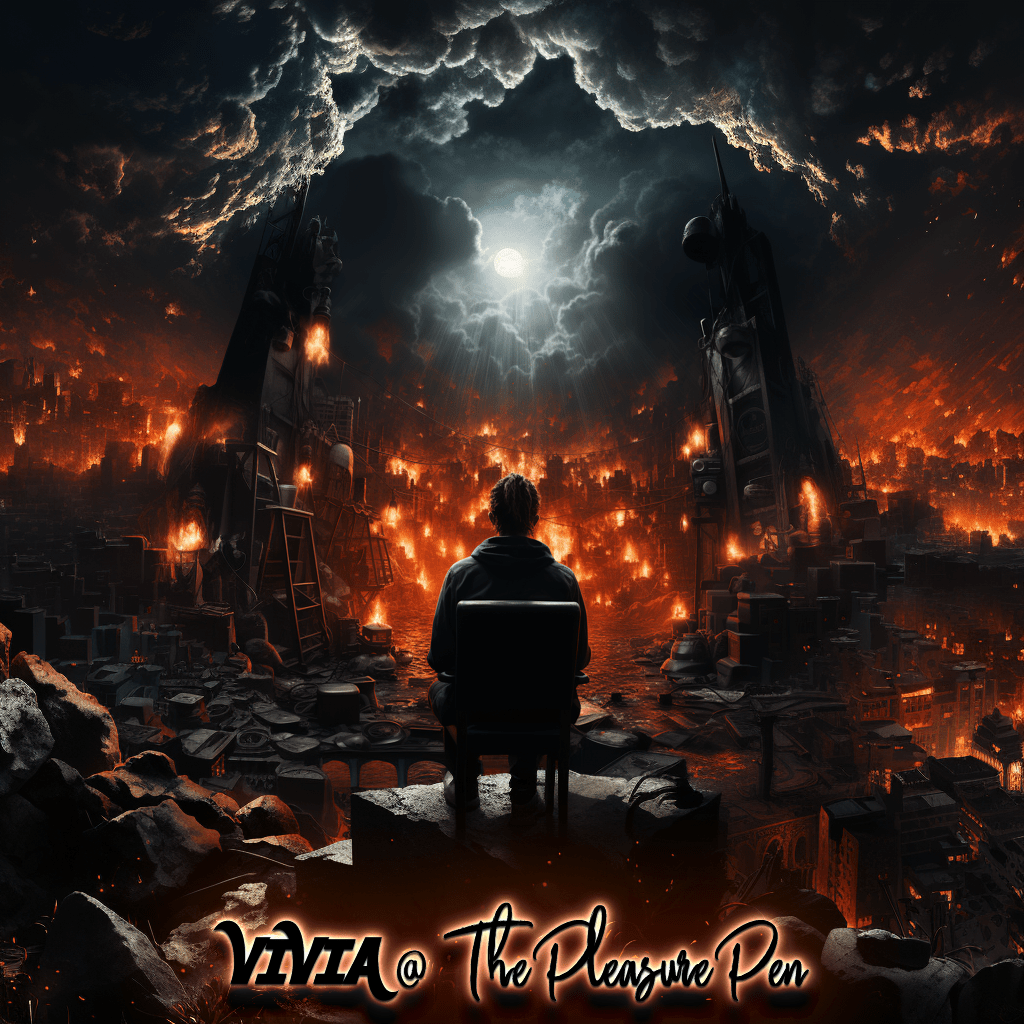In this highly detailed, post-apocalyptic animated image titled "Vivia at the Pleasure Pen," depicted in black cursive font at the bottom, we see a man sitting in a chair facing away from us. He wears a black hoodie and gazes out toward a scene of massive devastation. Surrounding him are large, blackened, and gray buildings, partially collapsed with scattered debris and pervasive fires emitting orange flames. The haunting ambiance is accentuated by blackened objects, burnt remnants, and small square-like structures. Prominent on either side of the man are two towering, charred structures with flames licking their edges. Above the scene, the sky is filled with imposing gray and black clouds, parted by an opening through which a luminous full moon shines, its light casting an eerie glow on the destruction below. The overall atmosphere is dark and somber, amplified by the gray clouds tinged with orange from the rampant fires, creating a chilling, nightmarish landscape.